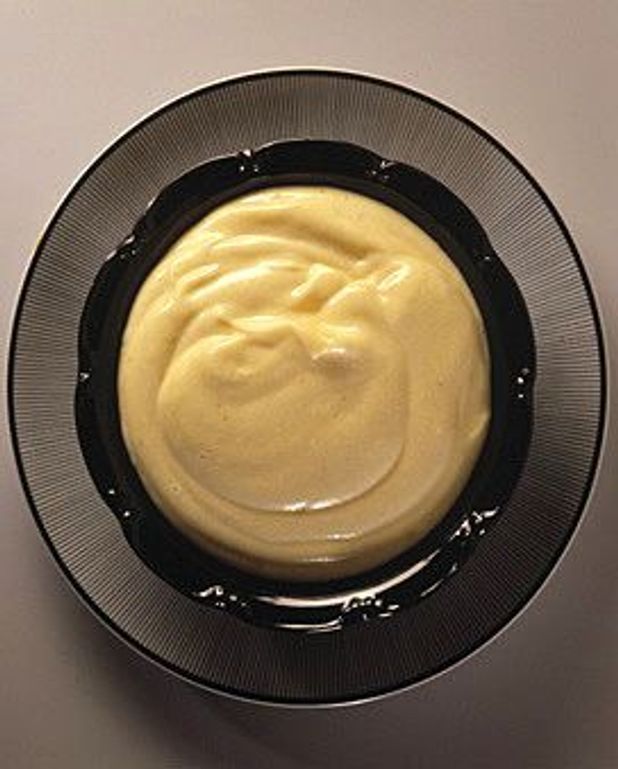This image features an overhead view of a shiny black bowl with a thin black rim, sitting on top of a ridged, black-rimmed plate. The bowl contains a smooth, light yellow substance that could be custard, pudding, or mustard, characterized by its creamy texture and semi-circular lines swirling towards the center. The interior of the bowl is glossier compared to its edges, and the background gradient transitions from dark mocha at the bottom to light brown at the top. The bowl and plate occupy the majority of the image, and there are no text or other elements present in the scene, only the bowl of yellow sauce prominently displayed.